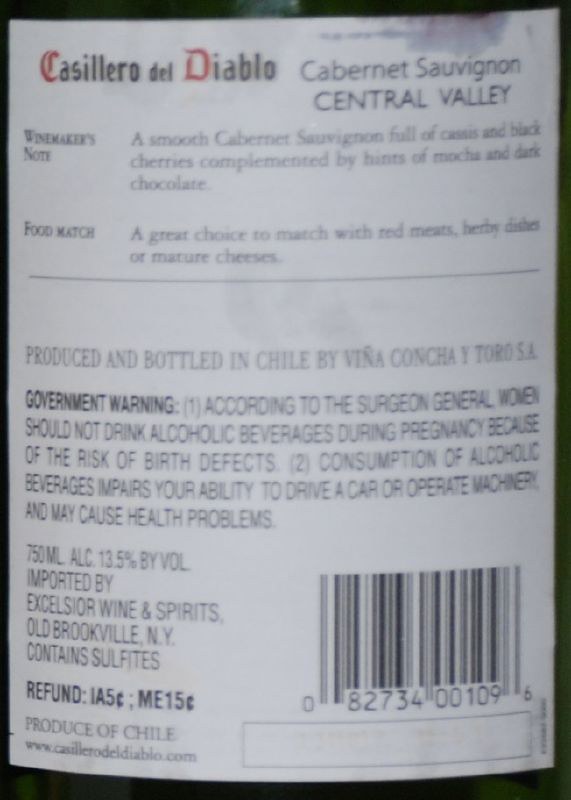The label on the side of a wine bottle is expertly detailed and prominently displays the designation "Casillero del Diablo," a Cabernet Sauvignon from Central Valley. The name, written in Spanish, features ornate red lettering for both the "C" in "Casillero" and the "D" in "Diablo," contrasting the primarily black text used elsewhere on the label. Directly beneath the name, the label reads "Wine Maker's Note," followed by a description of the wine: "a smooth Cabernet Sauvignon full of" — though one word is illegible due to smudging. The description continues, highlighting flavors of "black cherries complemented by hints of mocha and dark chocolate." Further down, you will find the "Food Match" section, which suggests that this wine pairs excellently with red meats, herby dishes, or mature cheeses. The label also includes the note, "Produced and bottled in Chile," affirming its origin. At the bottom of the label, mandatory information such as a government warning, details about the importer, refund information, website, and a UPC code are listed.